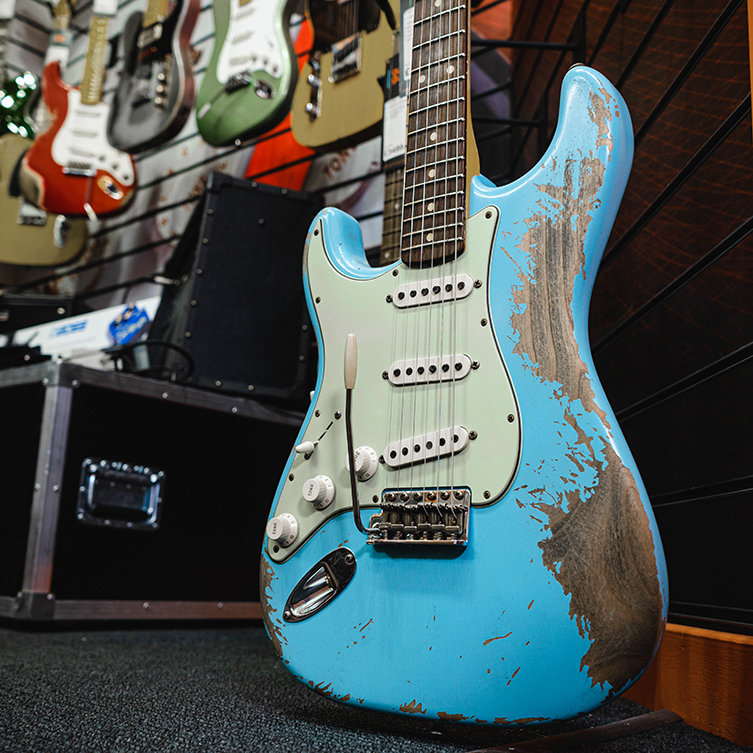This is a photograph of a vintage electric guitar prominently placed in the foreground of a guitar shop. The guitar, which stands upright, features a light blue body with significant paint wear, exposing the underlying wood grain in numerous spots. The wear and tear suggest that it has been well-used, contributing to its antique appearance. It boasts three white knobs situated on a white panel beneath its six strings, characteristic of traditional electric guitars such as a Fender. In the background, you can see a black wall adorned with at least five or six electric guitars hanging, adding depth to the scene. There is also a black guitar case or possibly a monitor visible, though it is somewhat indistinct. The overall ambiance of the shop and the condition of the featured guitar together create a nostalgic and well-worn aesthetic.